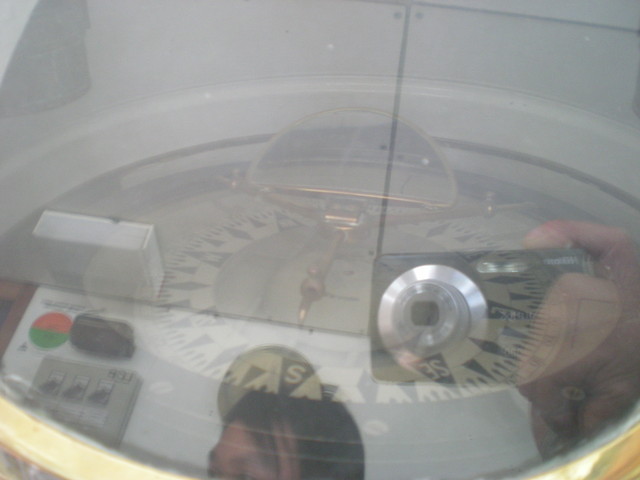The image depicts a complex reflection, primarily showing part of a woman's head with black hair situated in the bottom portion. It appears that she might be looking into the white cavity of a top-load washing machine. Superimposed over this scene is the reflection of a person holding a small digital camera, which casts an overlay of two squares onto the glass. Within the reflective surface, there is a compass-like dial featuring a reversed 'S' in a black triangle. To the left of this dial, two dots—one red and one green—are visible, alongside a black dial. Additionally, various rectangular boxes appear in the image: a gray box is located in the bottom left corner while other faint and fuzzy colors blend into the reflection, including touches of gold in the bottom corners. In the center of the image, there is a sunken half-circle component, which seems to be part of the watch or dial face, contributing to the overall intricate and layered reflection.